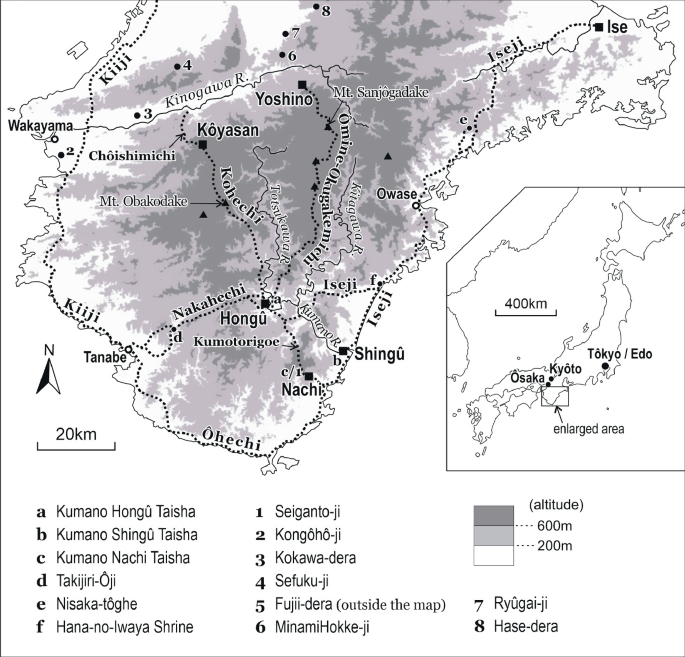The image portrays a detailed, drawn map of a region in Japan, specifically situated below Osaka, featuring various recognizable places and landmarks. The map is predominantly rendered in shades of black, white, and gray, with some elements accentuated in purple. Prominent locations such as Tokyo, Wakayama, Kumano Hongu Taisha, and Koyasan are clearly marked. Additionally, the map includes areas like Kumano, Tajiri, Misaka, and Hana no Iwana Shrine. 

An elevation key is present at the bottom-right, indicating altitude with white representing sea level, gray for 200 meters, and dark gray for 600 meters. Distance markers are visible, including a 20km bar on the left side and a scale conversion on the right side showing a corresponding 400km distance. The right side of the map features an enlarged section for more precise details. The entire image is set against a mostly white background, offering clarity in its depicted distances and terrain elevations.